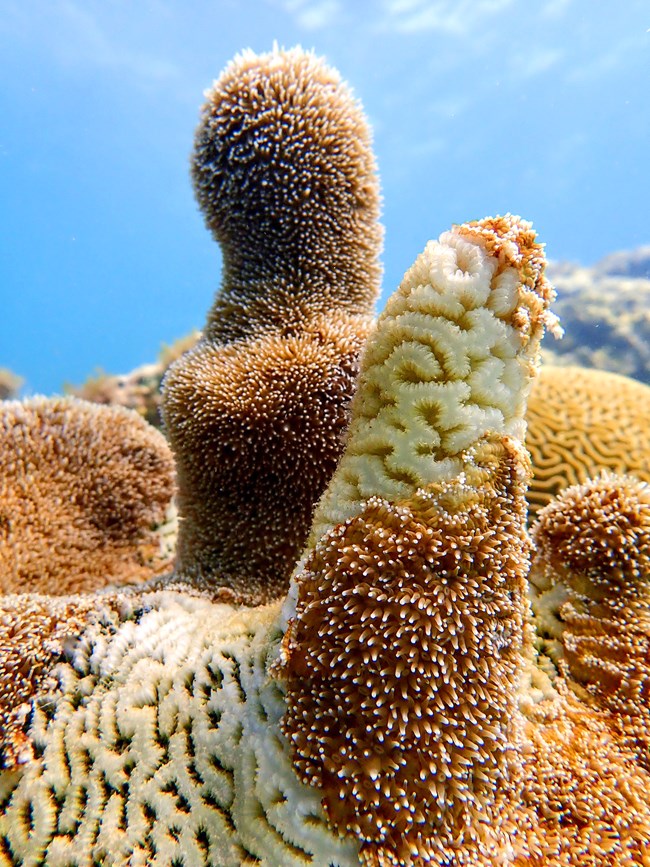This vibrant underwater photograph captures a lively scene within a shallow coral reef. The background features a striking turquoise blue, highlighting the clarity and cleanliness of the water. The foreground is dominated by multiple vertical coral formations that stand out with distinctive characteristics. One prominent formation is an orange-brown color, with lighter hues in the front and darker, more intense shades in the rear. The rear formation is adorned with fuzzy-looking nubs of coral, lending it a spiky appearance. Another notable formation in the foreground shares this texture, partially covered with similar spiky nubs and featuring a unique white section that boasts wiggly, brain-like curved lines.

Towards the right center, a coral formation has a brown, almost fur-like texture with white tips. This formation is about four inches tall and contributes to the intricate, squishy, and cotton-like visual texture of the scene. Above these formations, there are swirling white lines that resemble small worms, adding to the delicate complexity of the reef. The diverse color palette includes shades of brown, beige, tan, white, and yellow, enhancing the photograph's vividness and conveying the natural beauty of the coral ecosystem. 

Overall, the image captures the fascinating intricacy of living coral formations beneath the water's surface, making it apparent that it was likely taken by someone scuba diving and appreciating the vibrant underwater landscape. The natural structures, resembling stalagmites, combined with the bright background and detailed textures, highlight the dynamic and thriving environment of the coral reef.